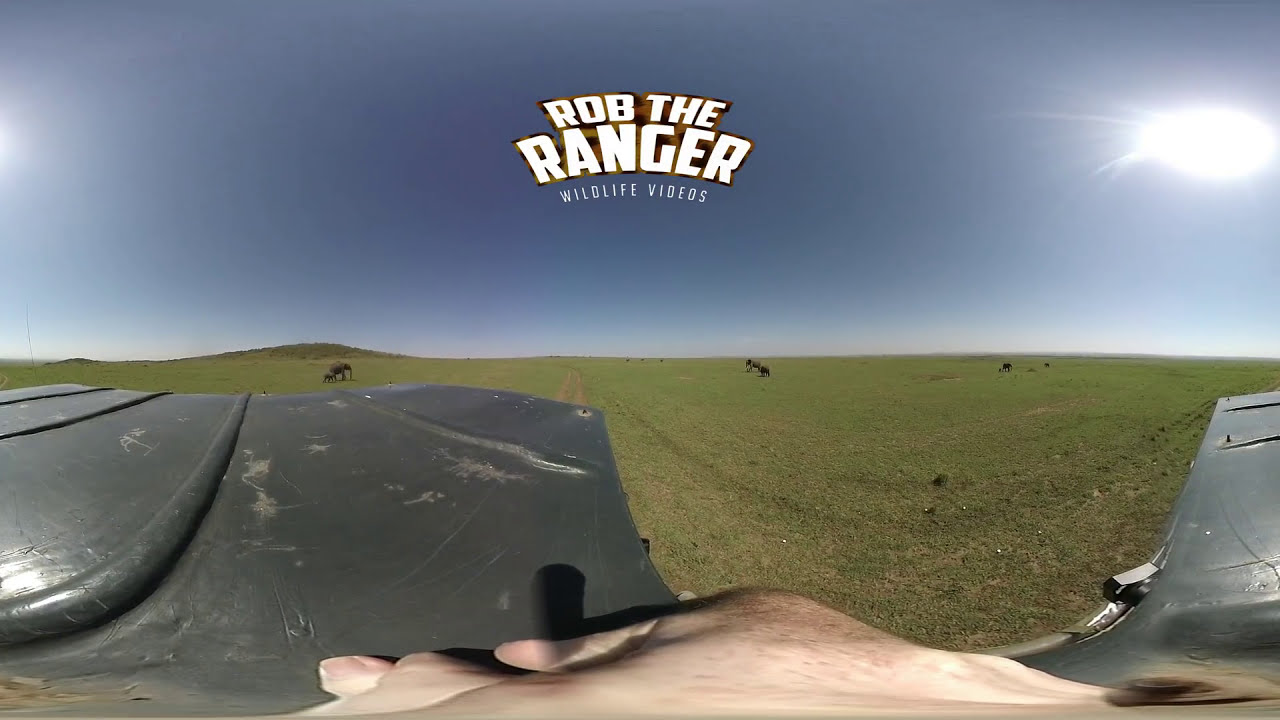The photograph captures a surreal, semi-abstract blend of two scenes, creating a visual effect reminiscent of a video game or an altered reality. The top half of the image portrays a gray-blue sky with bright white areas, particularly a silvery-white illumination in the top right corner, resembling the sun shining through clouds. Centered at the top, the text "ROB THE RANGER” is prominently displayed in large, semi-circular white letters with a dark background. Below it, in smaller white letters, reads "WILDLIFE VIDEOS."

The lower half of the image is divided into two blending pastures. Both sides feature a meadow with low grass where cows are seen grazing. The left pasture includes a cow grazing towards the center with some sort of gray, plastic-like object in the foreground. There's also a discernible human hand at the bottom, possibly holding a black knob. This foreground element extends into the right side, which mirrors the left but with a barrel distortion effect that emphasizes the curvature, making the scene look like part of an inception-styled composite. The right edge includes the same gray metal surface seen on the left. The overall composition with this blending and distortive filtering creates a unique, artistic representation, making the exact scenario slightly ambiguous but visually intriguing.